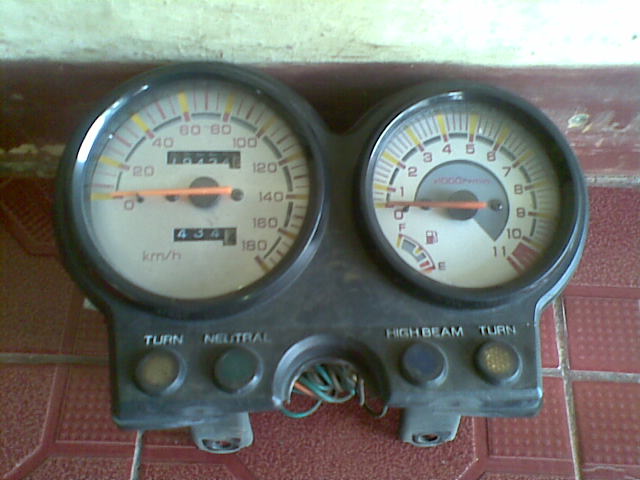This image showcases a detailed view of an automobile's instrument panel cluster that has been removed from its vehicle. On the left side of the cluster is the speedometer, featuring a white face and an orange needle currently resting at zero kilometers per hour. The speedometer is calibrated to display speeds up to 180 kilometers per hour. Adjacent to it, on the right side, is the tachometer, which also has a white face and is marked up to 11, indicating the redline. This tachometer is also at zero RPM and contains a small, integrated fuel gauge.

Below the main dials, the panel features various indicators and controls. On the left side, there is a section labeled "Turn" with an associated button below it, followed by a "Neutral" indicator with its corresponding button beneath. To the right of the tachometer, a "High Beam" indicator is present alongside its button. Additionally, this section has another "Turn" label with a button beneath it, which, along with the left turn control, signifies the left and right turn signals.

The instrument panel is entirely a cluster that houses the speedometer, tachometer, fuel gauge, turn signal indicators, neutral indicator, and high beam indicator, complete with corresponding controls, creating a comprehensive display for the vehicle's essential data and alerts.